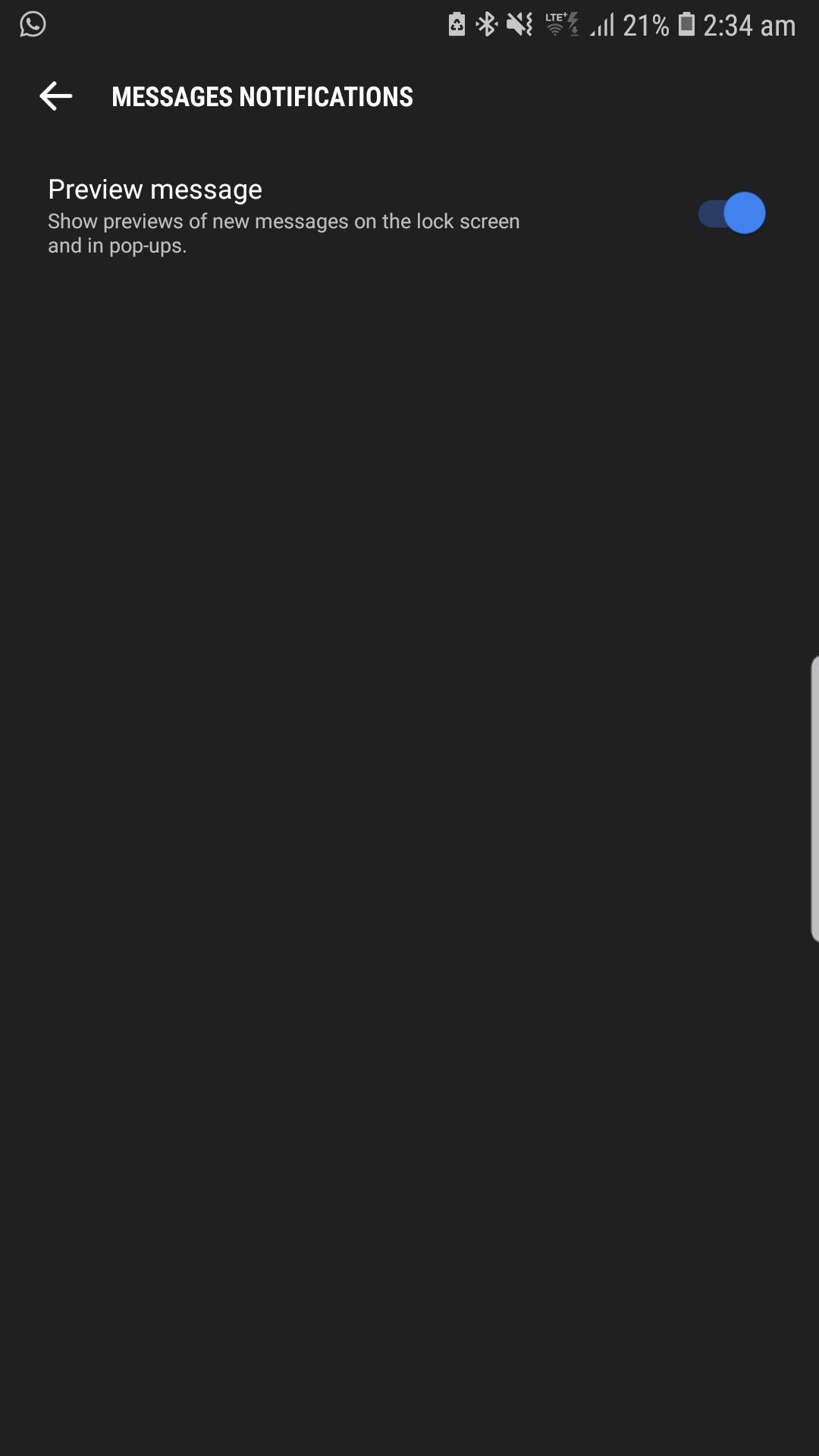This screenshot, set against a solid black background, captures a segment of a mobile device's settings interface at 2:34 AM, as indicated by the timestamp in the upper right corner. The top left corner features a white phone icon inside a circle, while the top right corner displays the Wi-Fi icon and a battery level at 21%.

Centered near the top, bold white text reads "Messages Notifications," with a left-pointing arrow adjacent to it. Directly below this, another line of bold white text states "Preview Message," which is accompanied by smaller white text explaining, "Show previews of new messages on the lock screen and in pop-ups." To the right of this descriptive text, a blue toggle switch indicates that the preview feature is currently activated.

The lower three-fourths of the screen remain entirely black, void of any additional text or icons. The screenshot effectively highlights the settings options for message notifications, particularly focusing on the ability to preview messages on the lock screen and in pop-up notifications, with the feature presently turned on as shown by the blue toggle.